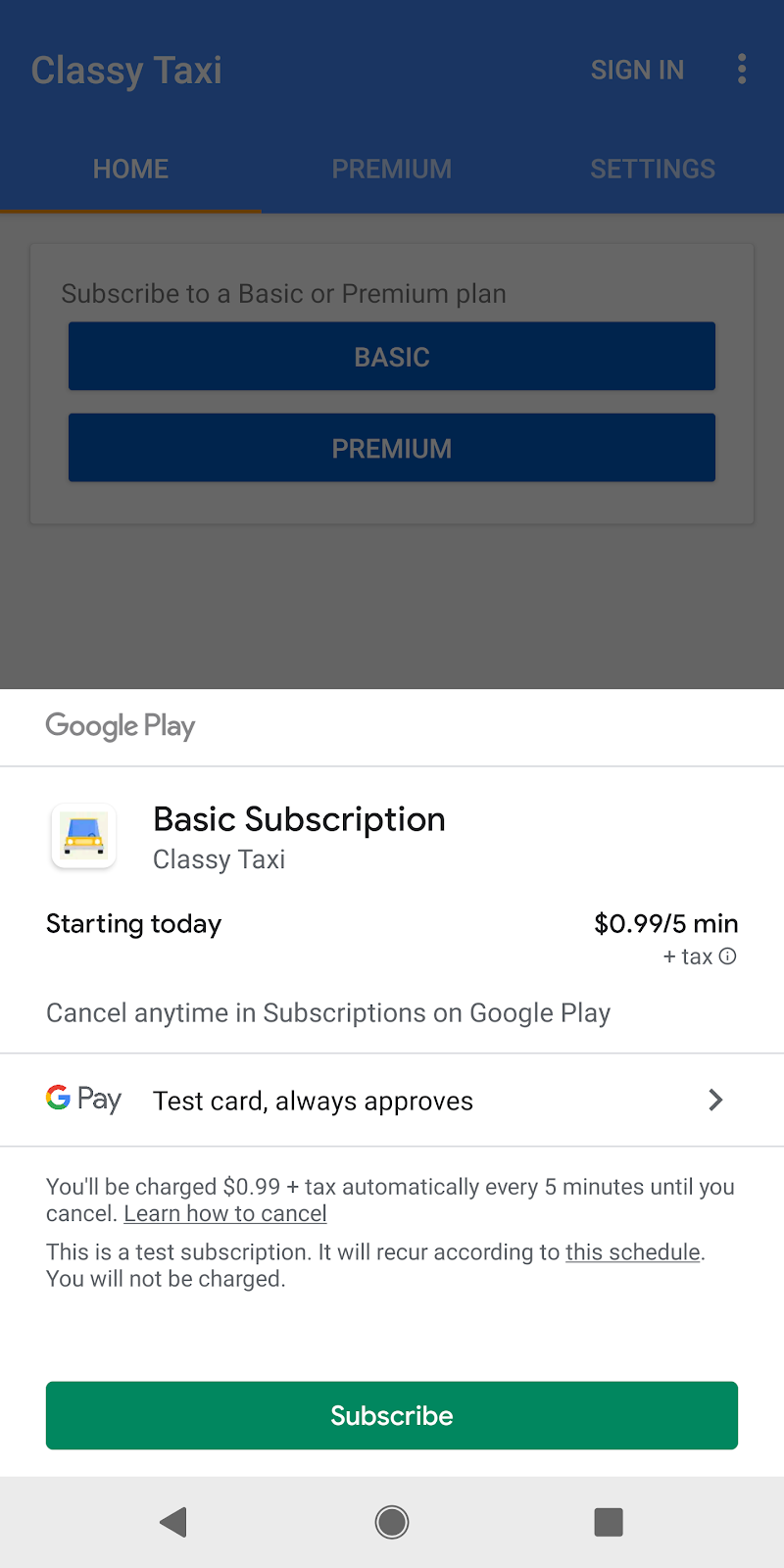The image depicts a digital interface with an overlay pop-up that partially obstructs the bottom half of the main screen. The main screen has a subdued, grayish tone indicating it is inactive. At the top, a prominent blue tab spans horizontally with the words "Classy Taxi" in white font on the left, and "Sign In" along with three dots on the right. Below this tab, three navigation features are evenly spaced: "Home" to the left, "Premium" in the center, and "Settings" on the right.

In the middle of the main screen, a centered gray box maintains the white background and reads, “Subscribe to a Basic or Premium Plan,” with both 'Basic' and 'Premium' capitalized. This box presents two large, white rectangular buttons labeled "Basic" and "Premium."

The pop-up overlay has a clean white background featuring a black Google Play logo at the top followed by a horizontal separator line. Below this line, there is an image that appears to be a taxi. Bold black text reads “Basic Subscription,” followed by "Classic Taxi" in a lighter shade. In a smaller black font, it states "Starting Today," and to the right, "$0.99 for five minutes plus tax." Additionally, gray text on the left mentions "Cancel any time and subscription on Google Pay." Below another line divider, it notes "GPA test card always approves," with an arrow pointing to the right. A green button labeled "Subscribe" is positioned at the bottom, ready for user interaction.